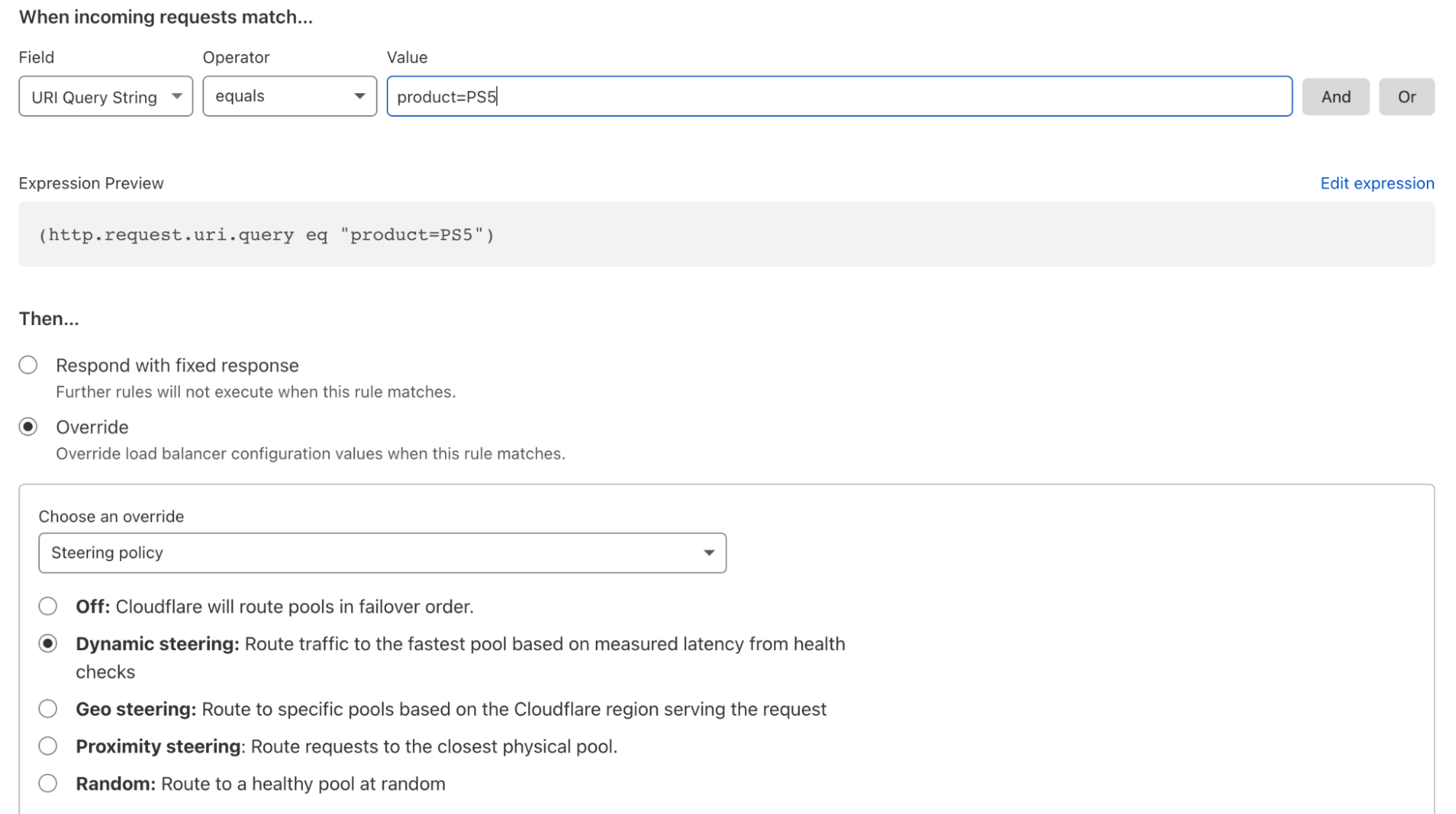In this detailed image, we observe a configuration interface with several sections. At the top, there's a header titled "When incoming requests match." Below this header is a field labeled "URL query string" where users can enter specific URLs. Adjacent to this, the field has an "Operator" dropdown set to "Equals," followed by an input box for "Value." Beside these fields are two buttons labeled "AND" and "OR" for combining multiple conditions.

The next section is titled "Expression Review," which contains a text box displaying some form of code. To the right of this box, there is a button labeled "Edit Expression" for modifying the existing code.

Following this, we find a section titled "Then..." which provides options for the system's response. There are two primary options: 
1. "Respond with fixed response," which has a note stating, "Further rules will not execute when this rule matches."
2. "Override," indicated by a dot in the override bubble. It contains a note that says, "Override low balance or configuration values when this rule matches."

Below the override option, there's a dropdown menu labeled "Choose an override," currently set to "Steering policy." Within this dropdown, several options are available:
- "Off": Cloudflare will route pools in failover order.
- "Dynamic Steering": Selected by default, it routes traffic to the fastest pool based on latency measured from health checks.
- "Geo Steering": Routes to specific pools based on the Cloudflare region serving the request.
- "Proximity Steering": Routes requests to the closest physical pool.
- "Random": Provides a final routing option.

The design of this page is predominantly white, featuring various text boxes and selection fields where users can input the necessary values or select options according to the configuration requirements.